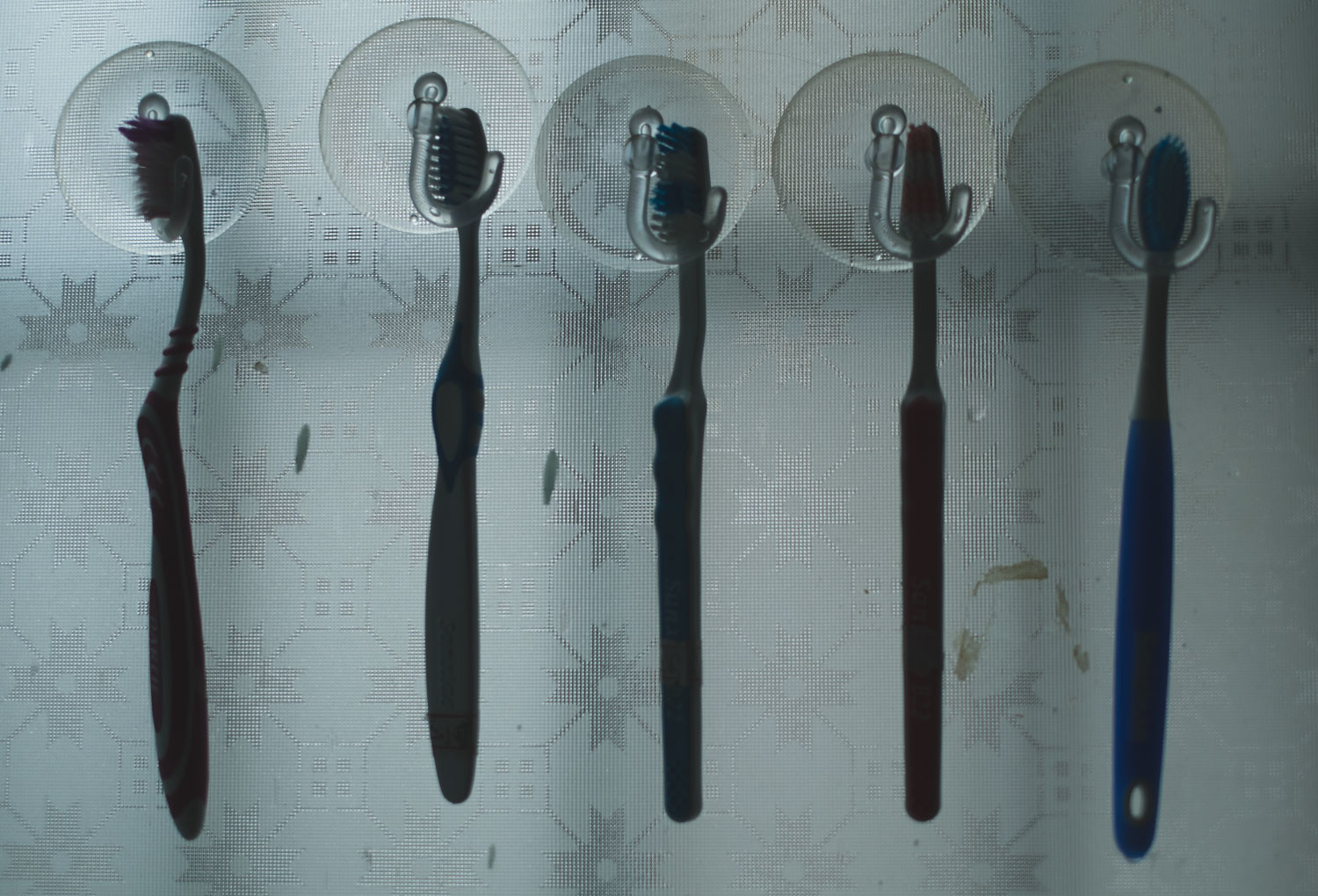This image depicts five toothbrushes hanging from transparent plastic hooks that are mounted on suction cups. The hooks adhere to a light gray textured surface, possibly glass, plexiglass, or ceramic tiles, adorned with intricate designs reminiscent of crosses and squares. The toothbrush handles point downward, while the heads are upright. Although the exact colors of the toothbrushes are hard to discern due to the dim lighting, the one on the far right appears to be royal blue. The remaining toothbrushes are indistinguishable in color but hang uniformly from the damage-free adhesive hooks. The scene is typical of a bathroom setting, potentially within a shower enclosure, adding to its utilitarian aesthetic.